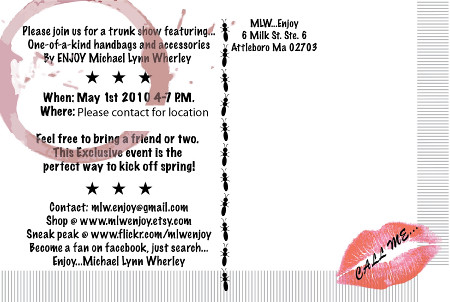The flyer is an invitation to a trunk show featuring one-of-a-kind handbags and accessories by Michael Lynn Worley. Prominently displayed at the top left is the text: "Please join us for a trunk show featuring one-of-a-kind handbags and accessories." Below this, it reads: "When? May 1st, 2010, 4-7pm. Where? Please contact for location. Feel free to bring a friend or two. This exclusive event is the perfect way to kick off spring." There are three stars separating various sections and contact information, offering details such as an email address (mlw.enjoy@gmail.com), shopping links (www.mlweenjoyetzy.com), and a sneak preview (www.flickr.com/mlweenjoy). Guests are encouraged to become a fan on Facebook by searching "Enjoy Michael Lynn Worley."

The right side of the flyer lists the address "MLW Enjoy, 6 Milk Street, Suite 6, Attleboro, MA 02703." A circular face graphic appears on the left under some of the text, and a line of ants runs down the middle of the image. Additional details include a red wine glass stain on the left and a striking lipstick kiss mark with pink lips in the bottom right corner alongside the words "Call Me" in black letters.